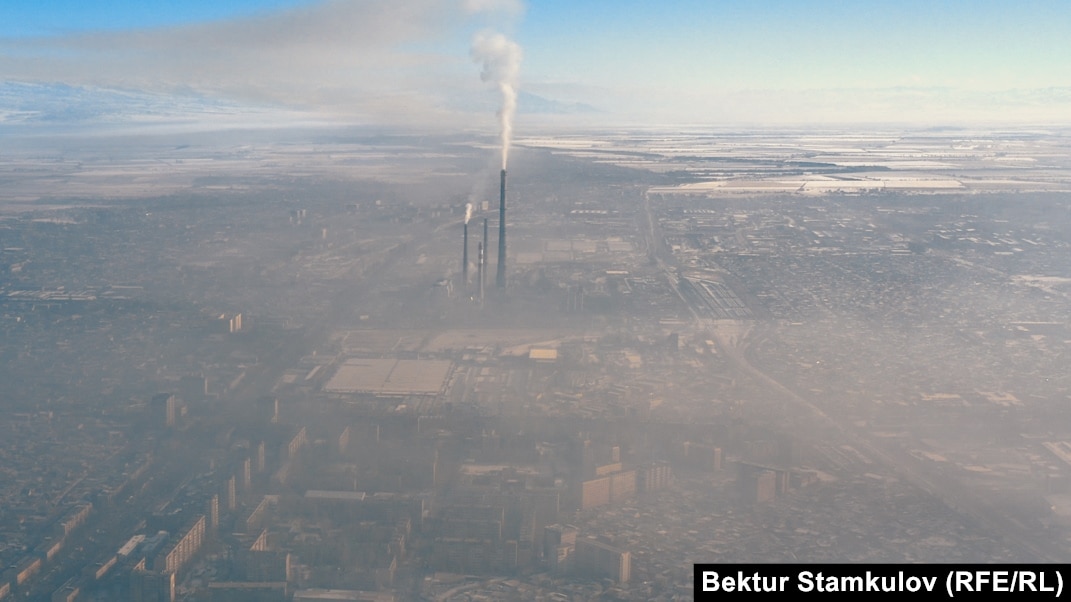The full-color photograph, taken during the day, captures an expansive aerial view of a hazy landscape that likely depicts a town or city. The top portion showcases the sky, transitioning from gray clouds on the left to a light blue expanse on the right. Just above the center of the image, three prominent smokestacks rise vertically; two are shorter, and the third, taller black smokestack emits a substantial plume of white smoke. The scene below is obscured by haze, making details difficult to discern, but a mix of brown tones suggests urban structures and possibly open ground dominating the midsection. In the bottom part of the photo, a road meanders from the lower left corner, curving up and right past the smokestacks, while another road seems to stretch horizontally across the image. In the bottom left corner, a black rectangular box with white text reads, "Bektur Stamkulov (RFE/RL)." The haziness intensifies towards the lower edge of the photo, further blurring the visibility of buildings and details.